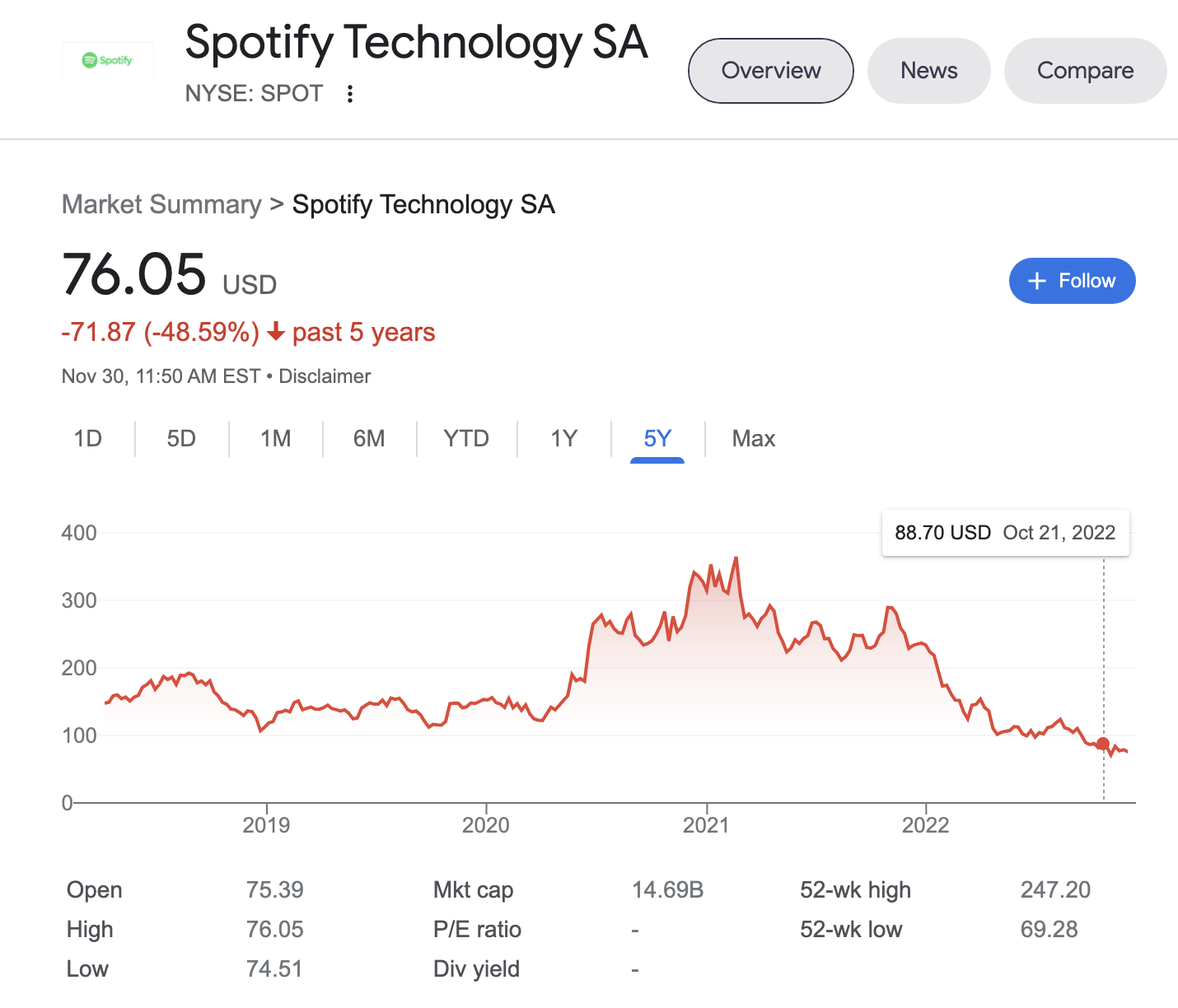The image displays Google's stock information page for Spotify, showing a detailed overview of the stock's performance. The current price of Spotify shares is $76.05 USD. The chart has been set to display data over a five-year period, starting from a value of $71.87 USD five years ago. The stock showed significant growth in 2021, but its value has subsequently decreased, with the data captured up to October 2022. Additional stock metrics are provided, including the opening price, daily high and low, market capitalization, 52-week high, and 52-week low. Notably, the Price-to-Earnings (P/E) ratio and dividend yield fields are blank. Overall, the stock's performance appears relatively stagnant over the observed period, indicating limited progress.